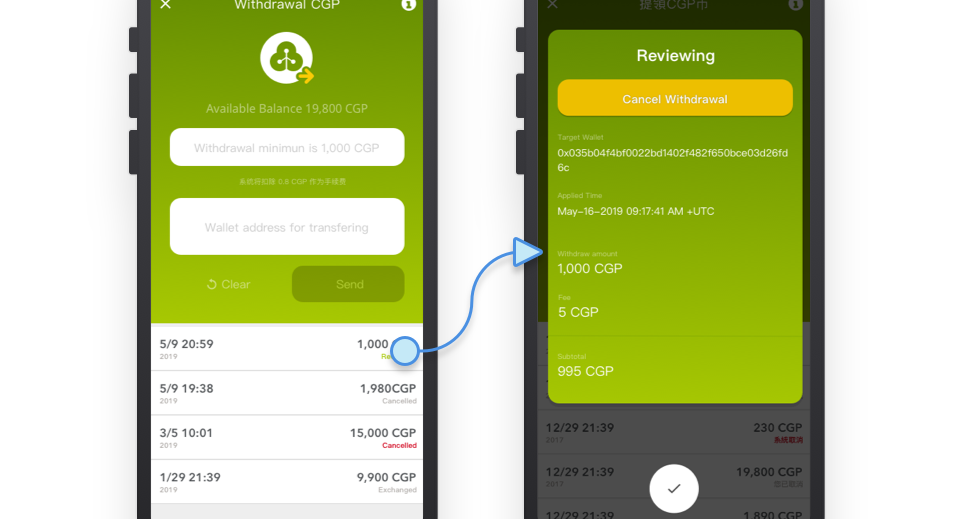The image depicts two cell phones side-by-side displaying a financial withdrawal interface. 

**Left Cell Phone:**
- At the top center, the title "Withdrawal CGP" is prominently displayed in white font.
- Below the title, there's a white circle containing an outline image resembling a tree.
- Beneath the circle, it states "Available Balance: 19.800 CGP" in clear text.
- Following that information is a white text input bar with a placeholder text indicating, "Withdrawal minimum is 1.000 CGP," written in a light greenish font.
- Further down, another text input bar is labeled with "Wallet address for transferring."
- At the bottom, four white rectangular boxes are lined up, each displaying dates and times. 

**Right Cell Phone:**
- On the screen, "1.000 CGP" is shown under "Withdrawal Amount."
- Notably, a blue arrow points from the top box on the left cell phone's screen to the corresponding "1.000 CGP" figure on the right cell phone screen, indicating a transaction detail or selection.

This detailed layout captures all the essential elements and user interface components present in the depicted withdrawal process on the cell phones.